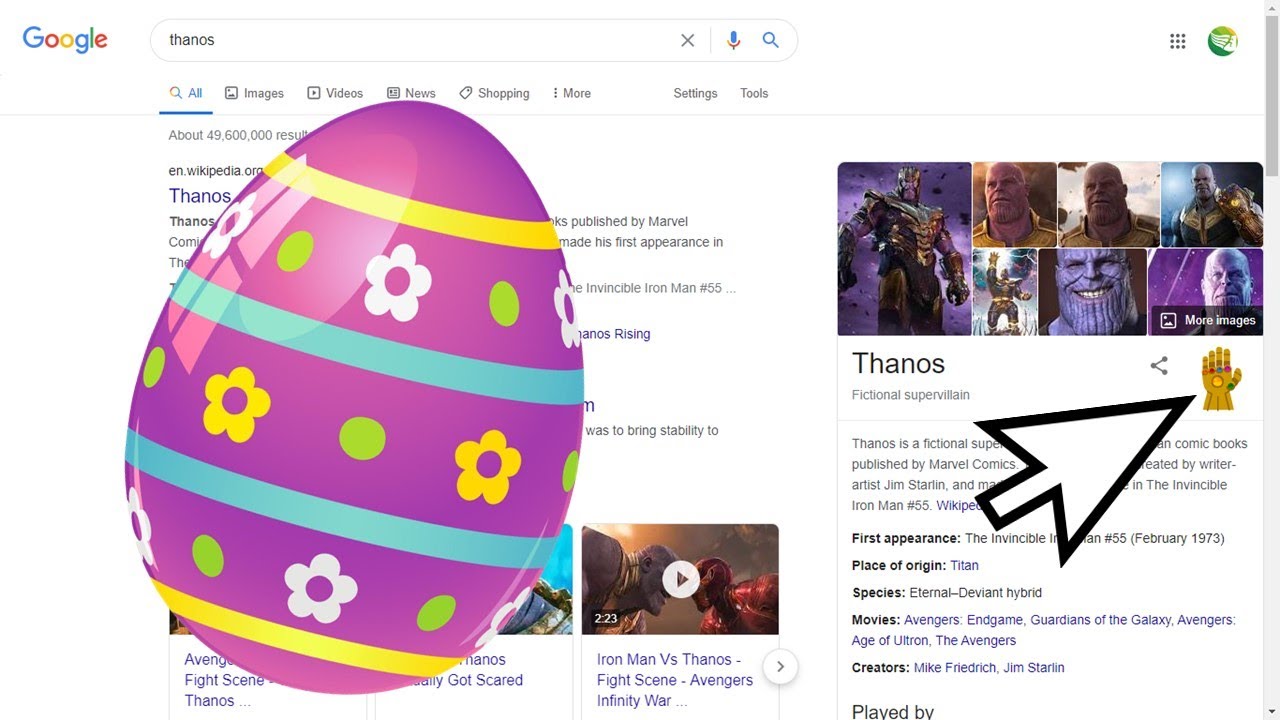On the Google search page, a large and intricately designed Easter egg takes center stage. The egg is predominantly purple and features multiple colorful stripes: one yellow, one turquoise, and one blue. The egg is further adorned with delicate white and yellow flowers scattered across its surface, adding to its festive look. In the background of this whimsical scene, the page reveals a search for "Thanos," a pivotal character from the Marvel Universe. A conspicuous, oversized arrow points directly to Thanos's hand, emphasizing a specific detail. Thanos, known as a mighty figure in the galaxy, becomes the focal point amidst the celebration of Easter, creating an interesting juxtaposition.